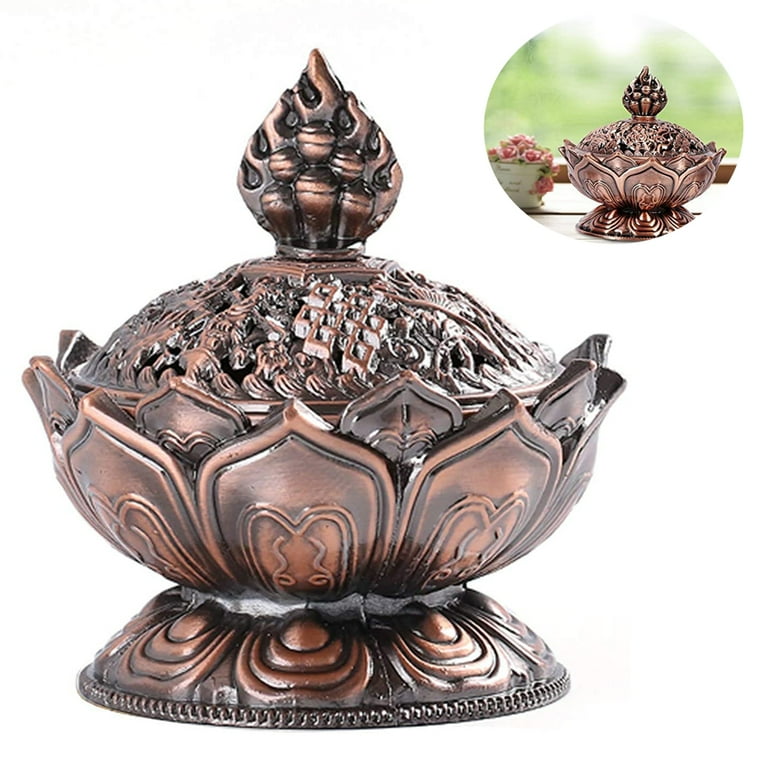This image showcases a detailed copper sculpture resembling a bowl with a base, intricately designed to mimic the shape of lily or lotus flowers. The bowl, made of metal and stained with a brown lacquer, holds various items including leaves and geometric shapes, with a flame-shaped decoration crowning the top. The primary view presents the sculpture against a white background, while an inset in the upper right corner provides a glimpse of it in a natural setting, placed near a windowsill with a green backdrop. The inset also reveals a small vase filled with flowers positioned to the left of the sculpture.